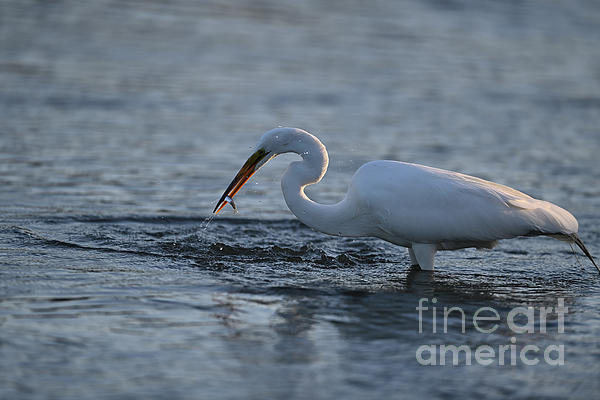This professional, horizontal photograph, likely sourced from Fine Art America, captures a white bird—possibly an egret—standing in calm, shallow water during the later part of the day. The bird, viewed from the side, showcases a long, slender, curved neck and an elongated orange beak, which contrasts with its pristine white feathers. Notably, the bird has a small blue fish clasped in its beak, with water droplets visibly trickling from the recent catch. The water around the bird appears dark blue-gray, with gentle ripples emanating from where it stands, suggesting recent movement. The scene is cast in a somewhat muted light, highlighting the serene and subtle interaction between the bird and its aquatic environment. The image is marked with the Fine Art America watermark in fine white letters at the lower right corner.